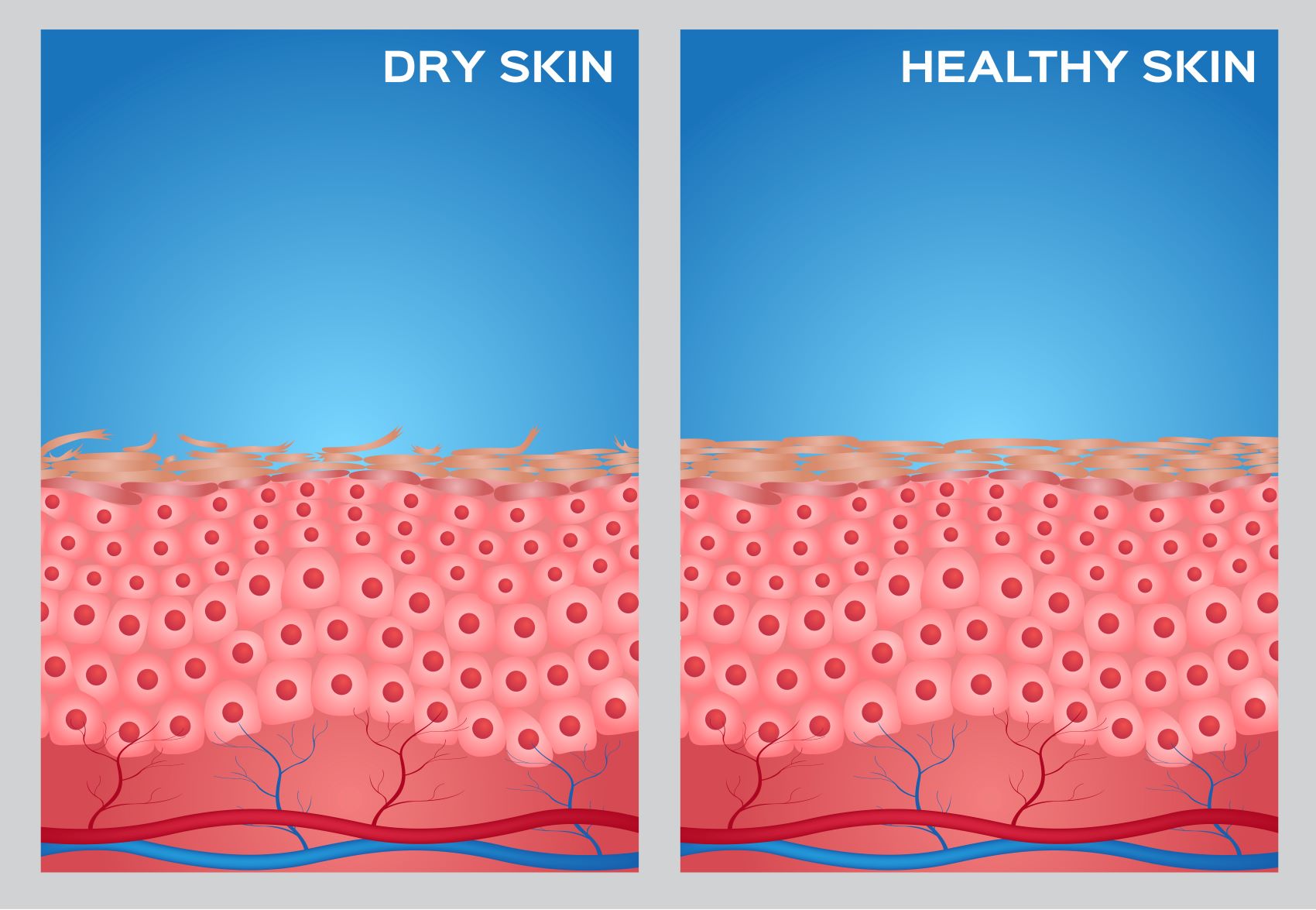The image features a detailed, side-by-side comparison of dry skin and healthy skin against a blue background, with "dry skin" labeled on the left and "healthy skin" on the right in white text. Both sections showcase the layers beneath the epidermis, highlighting veins and circulatory features in both light red and blue tones. The key difference lies in the outermost layer: dry skin has a rough, flaking surface with raised, crackly brown bits that are visibly peeling off. In contrast, healthy skin appears smooth, with interlocking, flat pieces that show no signs of damage or flaking. Despite their similar structure beneath the surface, the stark difference in texture and appearance of the outer layer exemplifies the disparity between dry and healthy skin.